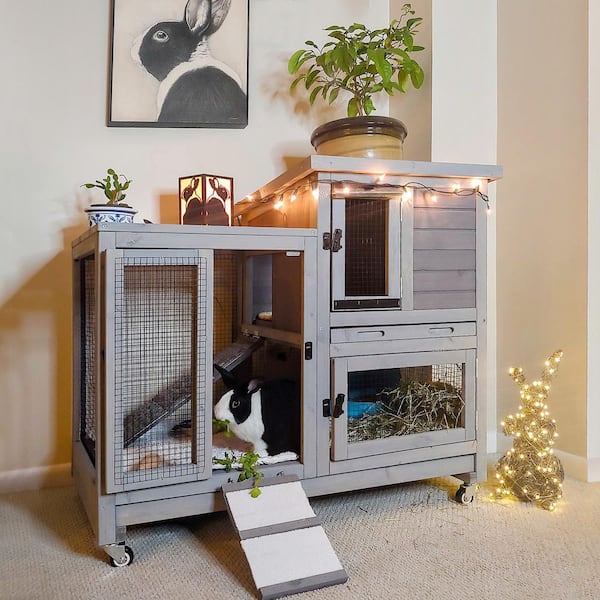The image showcases a professionally designed indoor rabbit enclosure that blends seamlessly with home decor. The cage, made of quality gray wood, resembles fine furniture and rests on black casters for mobility. It features a spacious, multi-level layout with interconnected sections. The left side has a two-tiered rectangular structure, including a lower hay-lined area with a blue food bowl, and an upper compartment accessed by a gray wooden ramp. The right side of the enclosure includes a large, mesh-wired door with an interior walkway for the rabbit to move freely.

Inside, a black and white rabbit enjoys a meal of lettuce. The cage is adorned with whimsical touches: white Christmas lights draped along the top and two potted plants alongside a candle featuring a rabbit motif. The setting is enhanced by neutral tan-colored walls and carpet, providing a cozy backdrop. Above the cage hangs an art print of the very same black and white rabbit, reinforcing the personalized nature of this charming space. Additionally, a decorative statue of a rabbit made from stiff rope or tumbleweed, also adorably lit with Christmas lights, stands beside the enclosure.